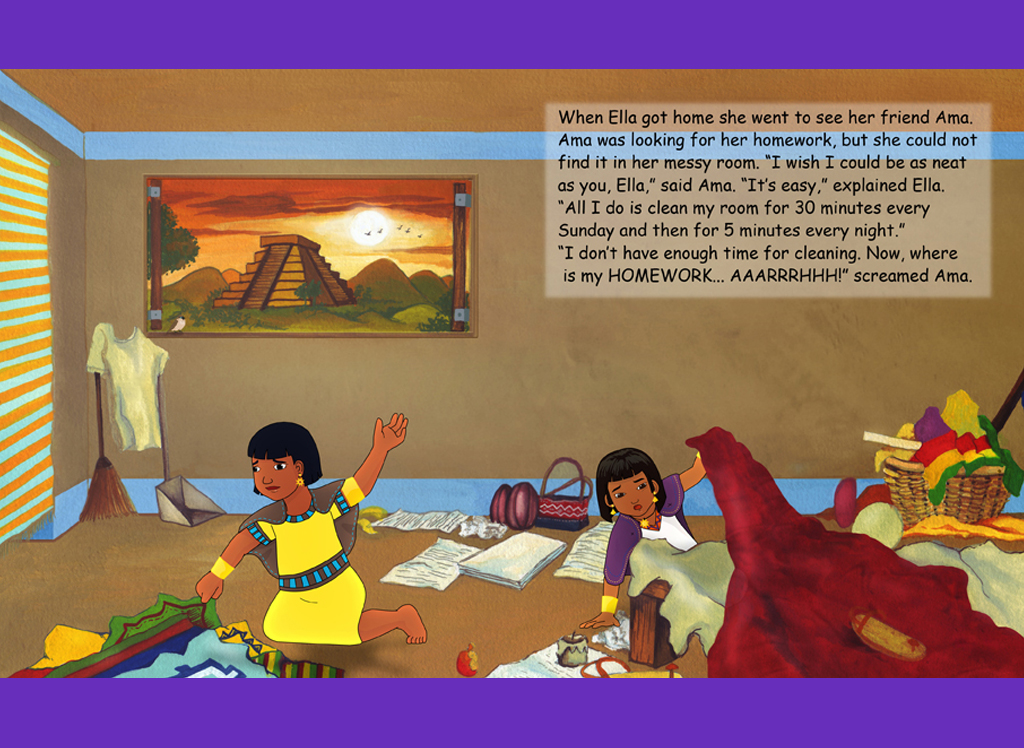This image is an illustration from what appears to be a children's book. It depicts a cartoon drawing of an ancient Egyptian-themed room, framed by thick purple borders at the top and bottom. The room is cluttered with clothes, papers, and blankets scattered around. On the left side, there's a window with a view of a pyramid, indicating the Egyptian setting. Two girls, dressed in Egyptian-style outfits, are present in the room. One girl, barefoot and wearing a yellow dress with a blue belt, has her arm raised. The other girl, wearing a purple top, is holding a large brown blanket. To the right, there is a basket full of clothes and a picture of a pyramid on the wall in the background. The text in the upper right corner reads: "When Ella got home, she went to see her friend, Amma. Amma was looking for her homework but could not find it in her messy room. 'I wish I could be as neat as you, Ella,' said Amma. 'It's easy,' explained Ella. 'All I do is clean my room for 30 minutes every Sunday and then for five minutes every night.' 'I don't have enough time for cleaning. Now where is my homework? Argh!' screamed Amma."